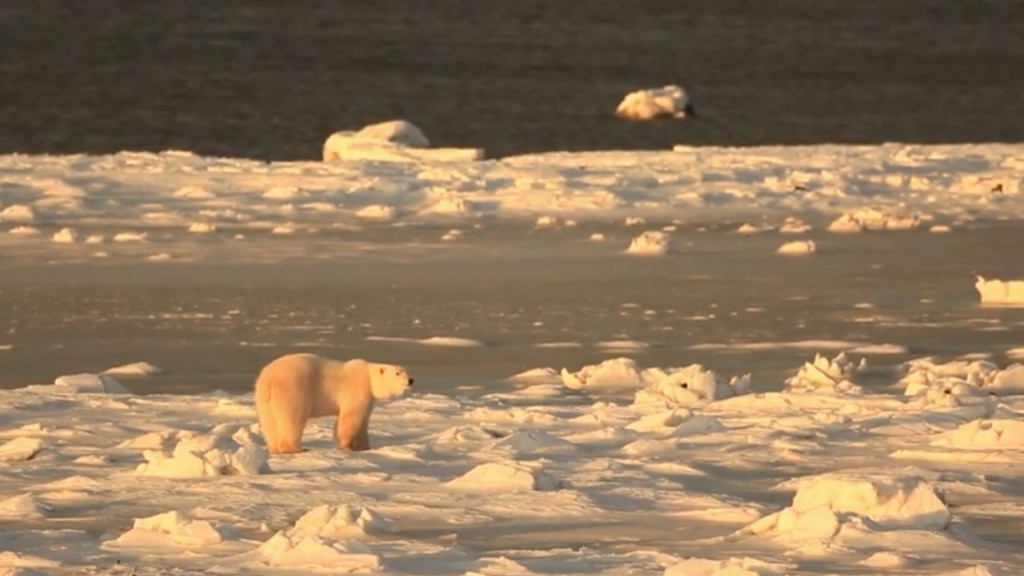In this striking photograph, a lone polar bear, primarily white with a hint of orange-beige fur along its back, stands on all fours against a backdrop of melting ice and snow. The foreground reveals ice that is rapidly melting, with slushy patches and small floating icebergs scattered around. The polar bear is positioned towards the left of the image, moving towards the right, starkly contrasting against the relatively flat and sparse snow. In the background, dark water dominates the scene, suggesting significant ice melt and the encroachment of the sea into formerly solid ice territory. The overall atmosphere of the image evokes a profound sense of loneliness and environmental change.